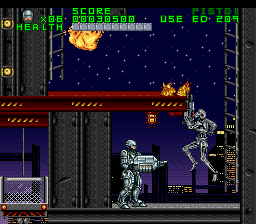In this video game scene set against a celestial night sky glittering with stars, a dramatic showdown unfolds. On the left, a blazing fireball streaks through the heavens. The action centers on a sleek, futuristic cityscape dominated by towering skyscrapers. One player, adorned head-to-toe in metallic gear and a sleek silver helmet, stands poised on a narrow metal beam high above the city. He wields a futuristic silver gun, aimed with precision at his airborne adversary. The second player, similarly clad in gleaming, high-tech armor, leaps through the air in a dynamic pose, creating a tense and visually striking scene. At the top of the screen, the game's score is displayed in bright green, accompanied by various other numerical and alphabetical indicators, adding to the immersive gaming experience.